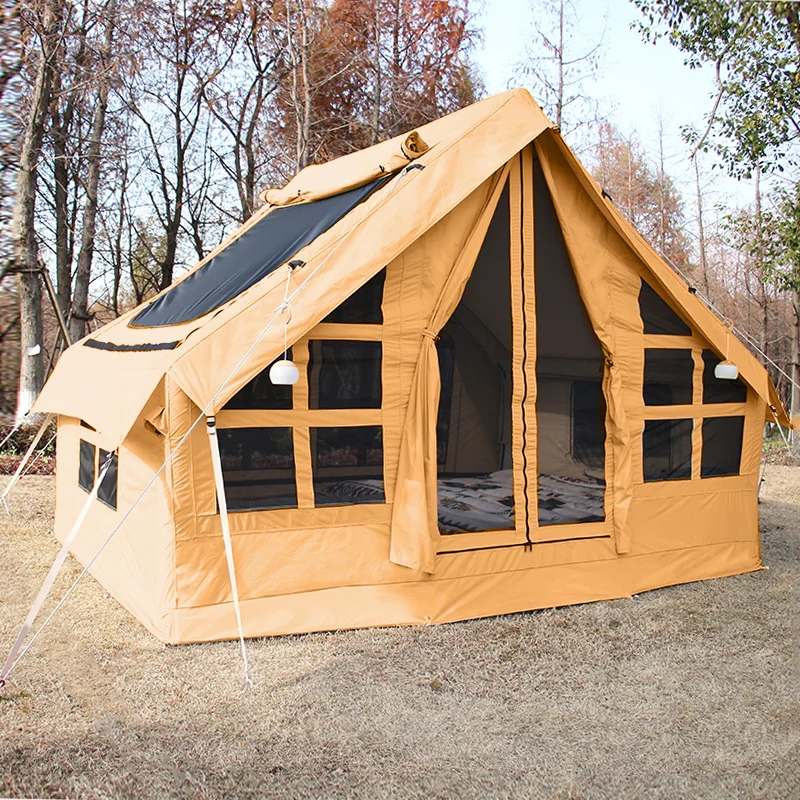The detailed photograph captures an outdoor scene, likely taken in the fall or early winter. The vertical, borderless image prominently features a large orange tent-like structure anchored to the ground on a patch of brown grass. The tent, which resembles a small home, is primarily orange-yellow with black mosquito netting that can be rolled up to let in light and air. The tent has multiple mesh windows and a large zippered door entrance, with white spheres, possibly lights, flanking the window areas. The interior of the tent is spacious and could accommodate up to six or more people; a flowery mat is visible inside. The backdrop reveals a blend of bare trees and others adorned with autumn-hued leaves, adding to the seasonal atmosphere. The sky above is partly cloudy, allowing some natural daylight to illuminate the scene, though the sun is not directly shining. The tranquil setting is enhanced by the quiet tree line in the distance, completing this serene outdoor tableau.